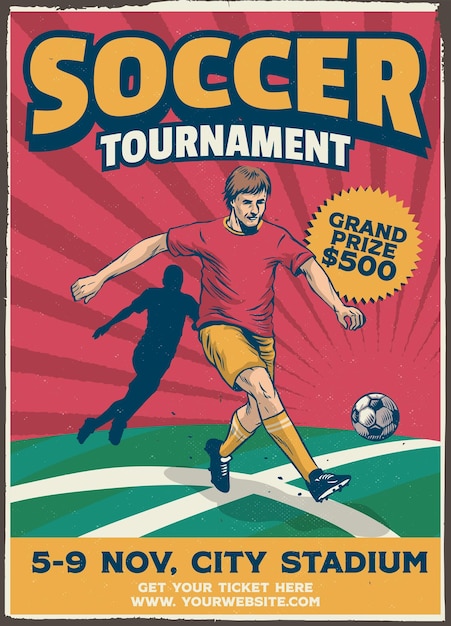This vibrant and dynamic soccer tournament poster features a color illustration centered around a male soccer player in the midst of an action-packed kick. Dressed in a short-sleeved red t-shirt, gold shorts, gold socks, and black and white soccer cleats, the player propels a soccer ball forward with great force. The background is characterized by dark red and light red rays that radiate outward, making the sky appear completely red, and suggesting an intense and exciting atmosphere. 

Enhancing the dramatic effect, a dark purple silhouette of another player looms behind the central figure, as if haunting or chasing him, adding a sense of urgency and competition. The green field beneath the players is marked with white lines, grounding the soccer action in a realistic setting.

Bold and eye-catching, the headline announces "SOCCER TOURNAMENT" with the word "Soccer" in striking orange letters and "Tournament" in simpler yet prominent white text, both set against a contrasting dark bluish backdrop. Below the action, a starburst graphic over the player's left arm highlights the grand prize, $500, in yellowish gold text.

At the bottom of the poster, a gold banner clearly details the event's specifics: "5 to 9 November, City Stadium" in black text, with an additional note directing spectators to secure their tickets at www.yourwebsite.com in smaller white font. The entire poster, possibly made to appear as if printed on metal with an artificially rusted edge, captures the excitement and intensity of the upcoming soccer event.